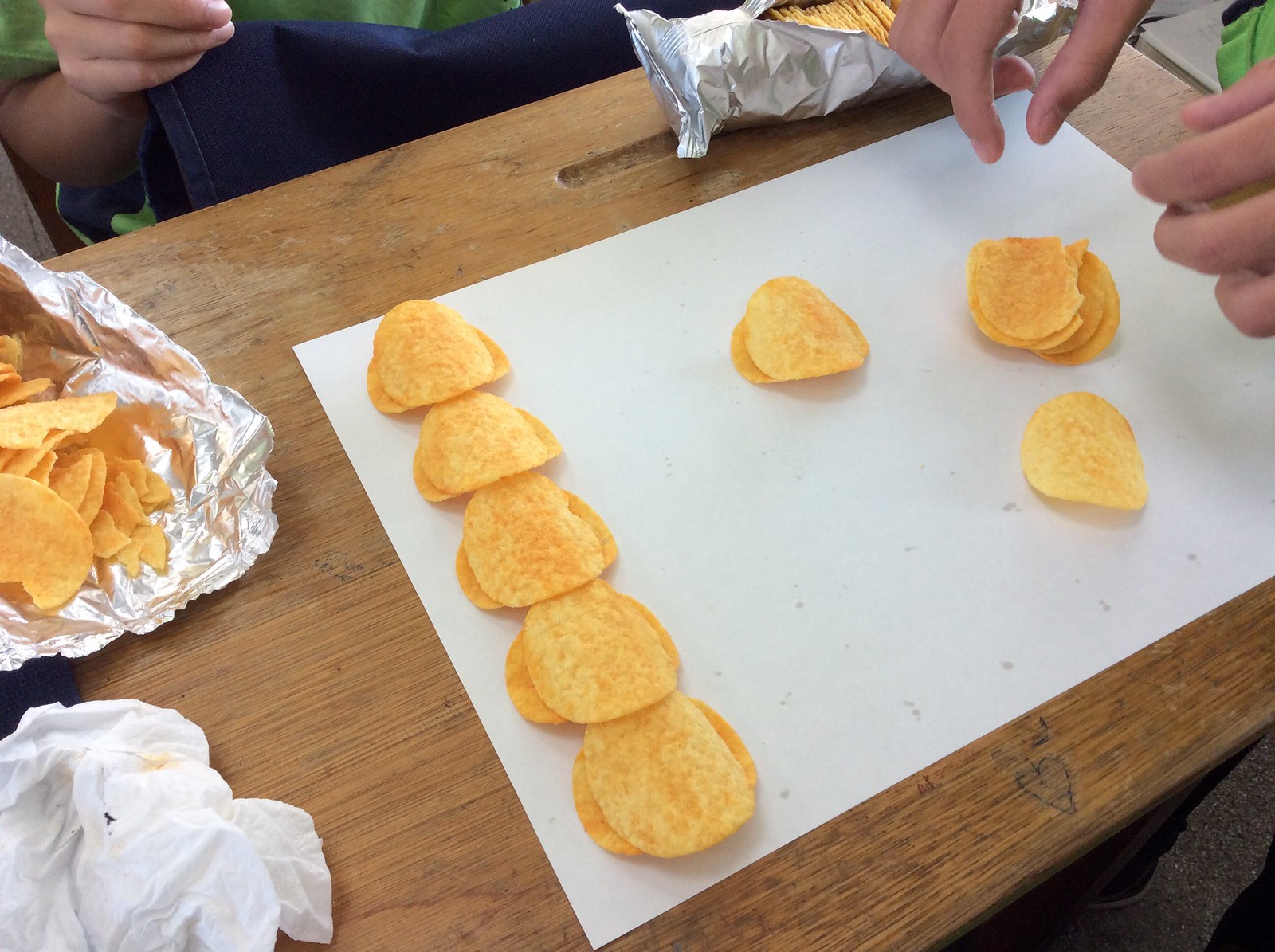The color photograph depicts a wooden surface, likely a table, viewed from a downward 45-degree angle. Central to the composition is a white sheet of paper situated on the table. Arranged meticulously on the paper, potato chips are organized in a line starting from the bottom left and moving diagonally to the back right before extending towards the bottom middle of the image. The chips are primarily stacked two high, with the bottom chips oriented left to right and top chips placed vertically.

In the upper right-hand corner of the photograph, a pair of hands appears, with the right hand adopting a pincer grip position, likely reaching to pick up one of the crisps. To the right, another small stack of crisps is noticeable, along with a couple of individual chips scattered nearby. Additionally, an open silver foil package of potato chips protrudes slightly into the frame from the left side, indicating the origin of the crisps.

A second person's presence is inferred from the partially visible right arm and hand at the back of the image, slightly cropped. This individual appears to be holding a navy blue napkin, possibly suspended or about to be placed on their lap, suggesting simultaneous engagement in the activity or preparation. The upper left-hand quadrant of the image also reveals a crumbled napkin and an observer's hand, identifiable by a green shirt sleeve, adding to the sense of collaborative effort or interaction.